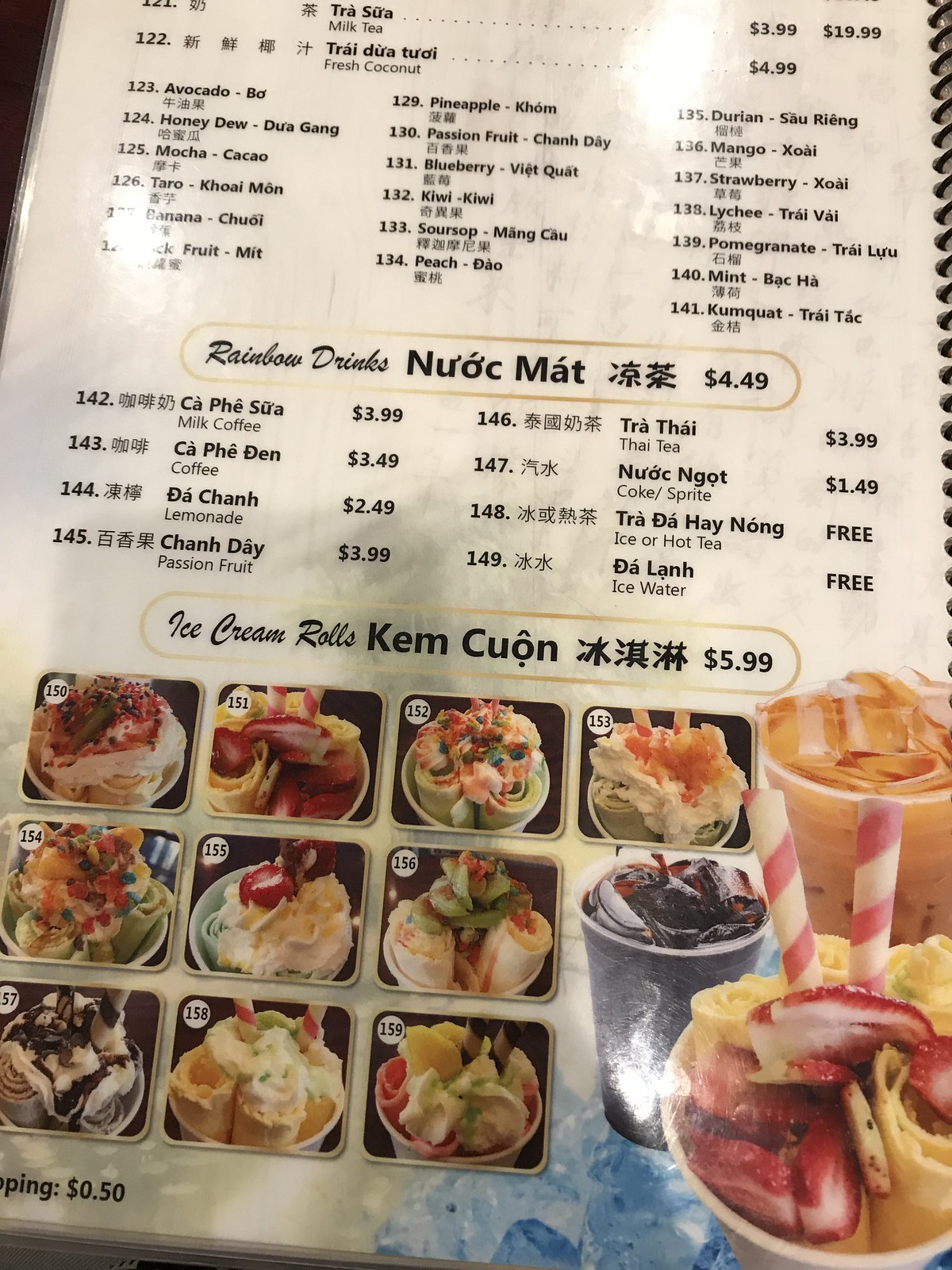This rectangular photograph captures a tilted menu, creating a perspective where the bottom appears larger than the top. The menu leans slightly to the right, revealing its multi-page nature, bound by a black metal spiral on the right margin. Printed on a white background, the menu features arrays of black text, showcasing both Asian characters and English descriptions. The listed items begin with "121 Milk Tea, $3.99," followed by prices in the range of $4.99 to $19.99. The offerings include diverse flavors such as "Fresh Coconut," "Avocado," "Pineapple," "Durian," "Honeydew," "Passion Fruit," and "Mango." Some items have additional descriptors and prices, for instance, "122 Fresh Coconut, $4.99" and "134 Honeydew, Duragon." The meticulous detailing of beverages continues, indicating an extensive variety available to patrons.